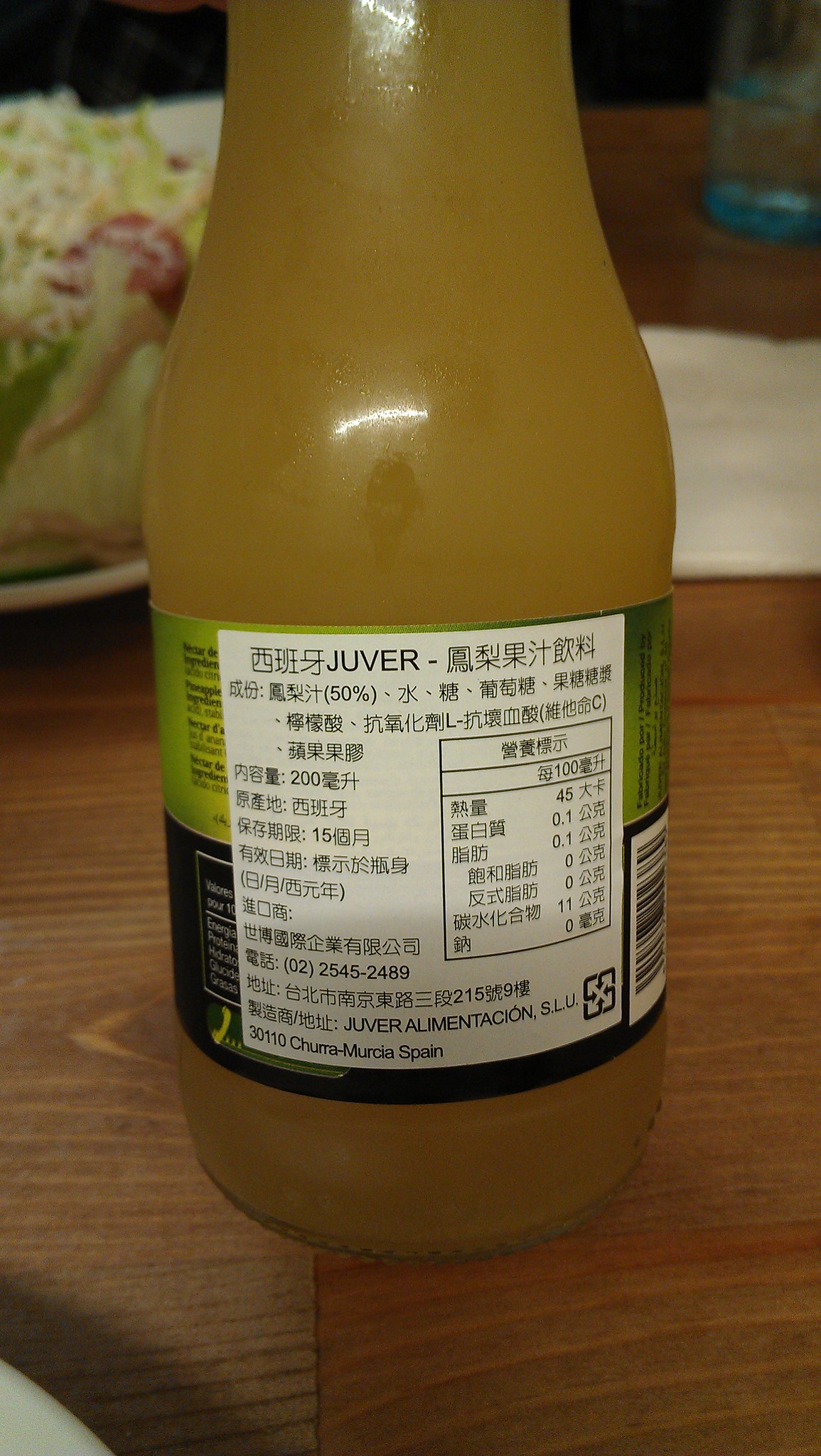The image captures a detailed scene of a wooden table setting. Centrally positioned at the bottom of the picture is a glass jar filled with a brownish, possibly apple juice-like liquid. The jar's label prominently features the brand name "Juver" and is adorned with various details in both Chinese and Spanish. The label has a white middle section with green sides and seems to include product-specific information, indicating 50% and 200 calories per serving, and it mentions Juver Alimenticon SLU, 3011 Chiramuria, Mauritius, Spain. The jar's top extends out of the frame.

In the blurred background to the left, a white plate is visible, holding what appears to be coleslaw, a sandwich, and potentially a yellow and red item resembling a Romano tomato. A small napkin is placed above the center of the plate. At the upper right corner, there's a glass of water with a blue bottom. The table itself is wooden with a pronounced wood grain running from left to right.